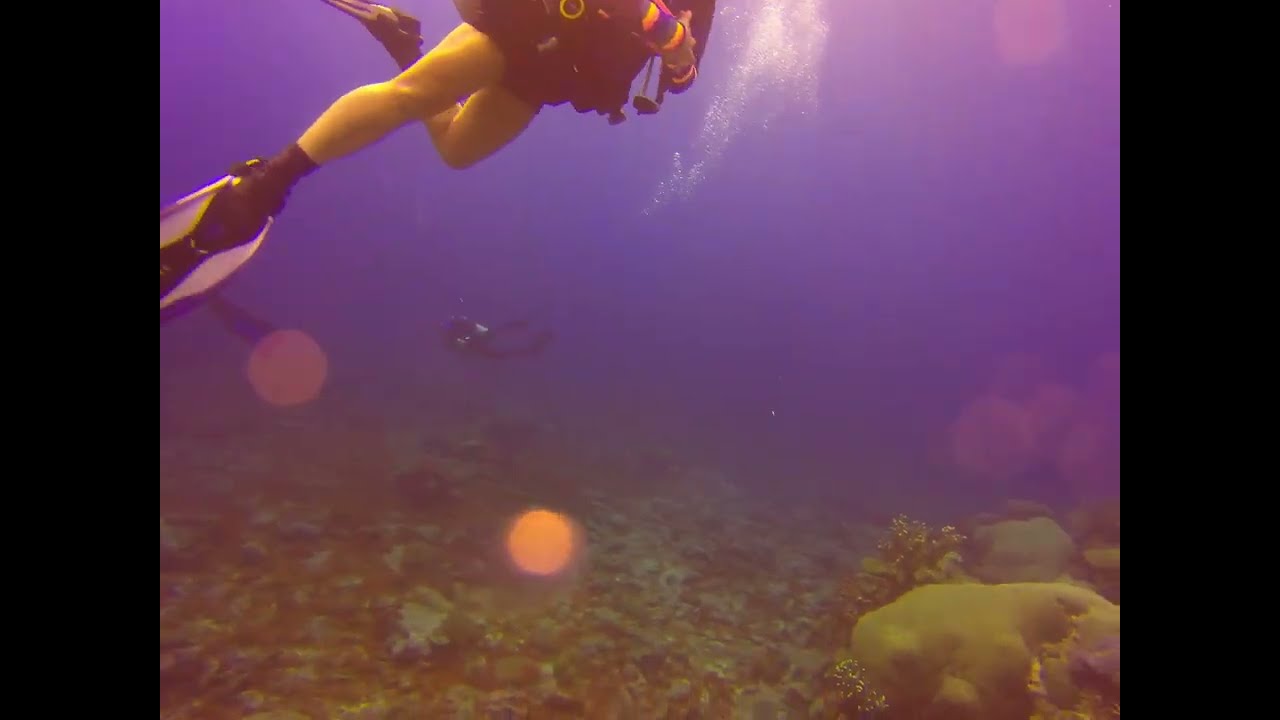In this rectangular, horizontal image, we are presented with an underwater scene bathed in an unusual spectrum of purples and pinks. The water is an ethereal blend of bluish-purple and pinkish hues, giving the scene a surreal quality. 

Dominating the upper left section of the image is a partially visible scuba diver, identifiable by their black flippers and yellow pants, and wearing a tight black top. Their head and shoulders are cropped out, revealing only from the chest down. This primary diver appears to have bare legs. Bubbles rise around them, enhancing their breathing action.

In the background, closer to the center of the image, a second scuba diver swims. This figure is further away and less distinct, primarily appearing as an outline, clad in mostly black gear. 

The lower portion of the image reveals the ocean floor, detailed with a coral reef that includes various corals and plant life in off-tan and brownish tones. The floor is rocky, with both large and small rocks scattered about, and minimal visible marine life, focusing the attention on the divers themselves.

The entire scene is framed with a black border on the left and right sides, but no border on the top or bottom, drawing the eye horizontally across the vivid, underwater tableau. Lights within the scene suggest it might have been captured by an underwater camera, lending further intrigue to this underwater adventure.